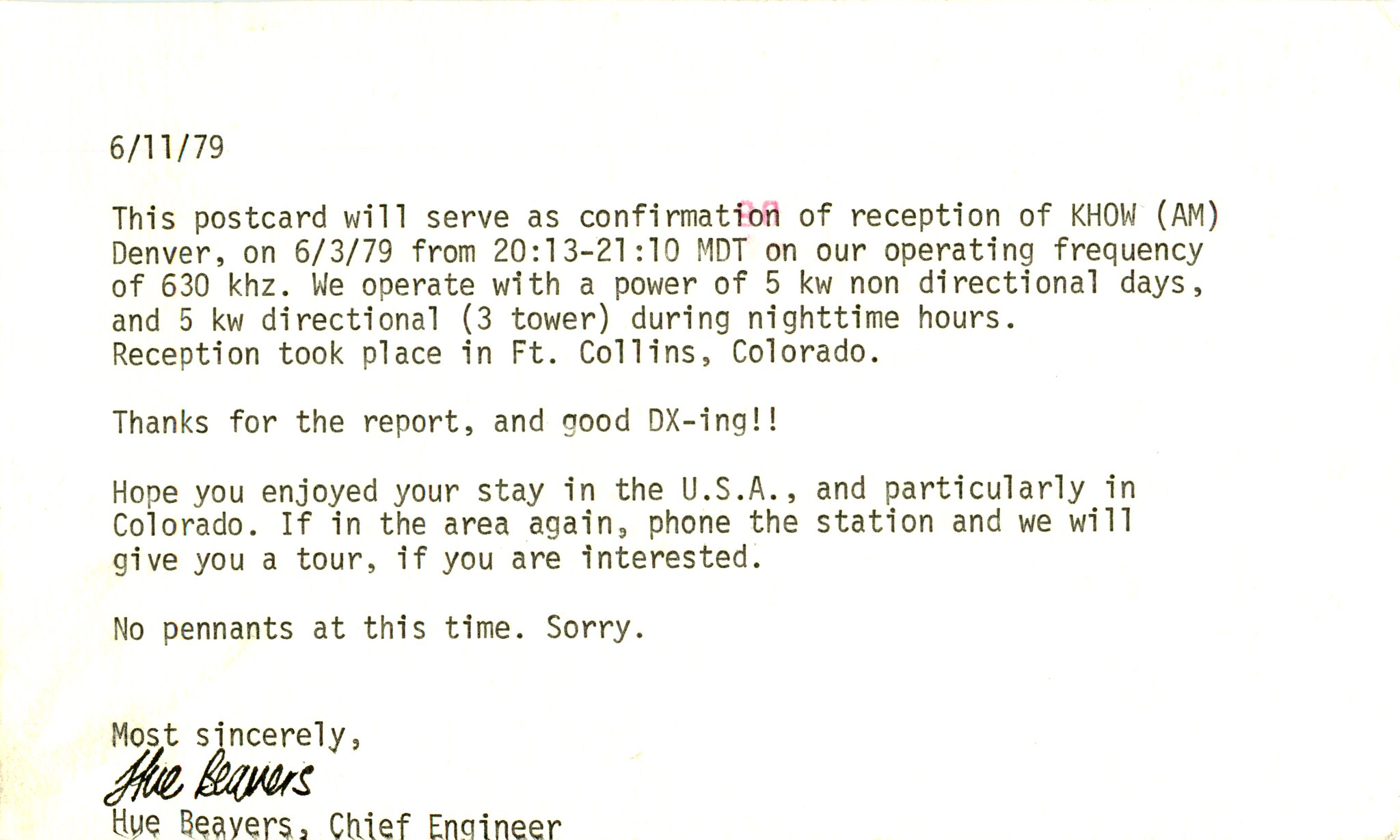This is an old white postcard dated June 11, 1979, with text appearing in a typewriter font. At the top left corner, it has the number "61179." The message on the postcard reads:

"This postcard will serve as confirmation of reception of KHOW AM Denver on 6-3-79 from 20:13 to 21:10 MDT on our operating frequency of 630 KHZ. We operate with a power of 5 KW non-directional during the day and 5 KW directional (three towers) during nighttime hours. Reception took place in Fort Collins, Colorado. Thanks for the report and good DXing. Hope you enjoyed your stay in the USA and particularly in Colorado. If in the area again, phone the station and we will give you a tour if you are interested. No penance at this time, sorry. Most sincerely, Hugh Byers, Chief Engineer."

The signature of Hugh Byers, the Chief Engineer, appears below this printed text.